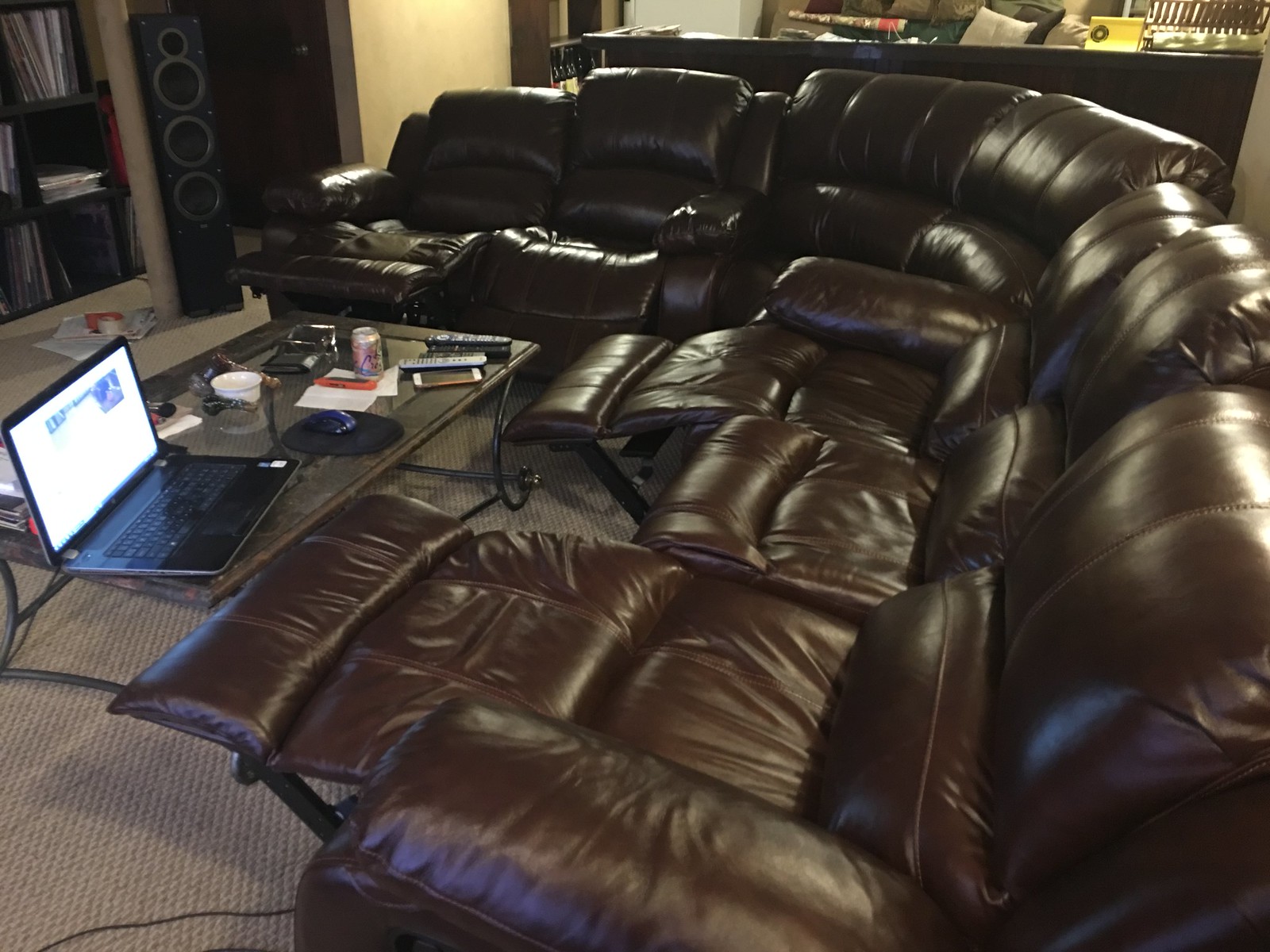The photograph captures the inviting interior of a living room primarily dominated by a brown leather sectional couch configured in a semicircle, giving each seat a recliner function. There are seven recliners in total, with the positions alternating between extended and retracted; the first, third, and last seats have their footrests up. A sleek glass coffee table with a metal base sits at the center of this arrangement, cluttered with everyday household items: a laptop with a white screen, a mouse pad, a Coca-Cola can, a La Croix water can, multiple TV remotes, a phone, and various other knick-knacks. The table is also surrounded by books and magazines. To the left side of the room, a large tower speaker with four protruding speakers and a possible record collection can be seen, while a dark brown wooden bar is partially visible on the right. Additionally, the backdrop features a half-height wall, suggesting the presence of another seating area just beyond the primary view. The recliners being raised and the visible cord imply that someone is about to vacuum underneath.